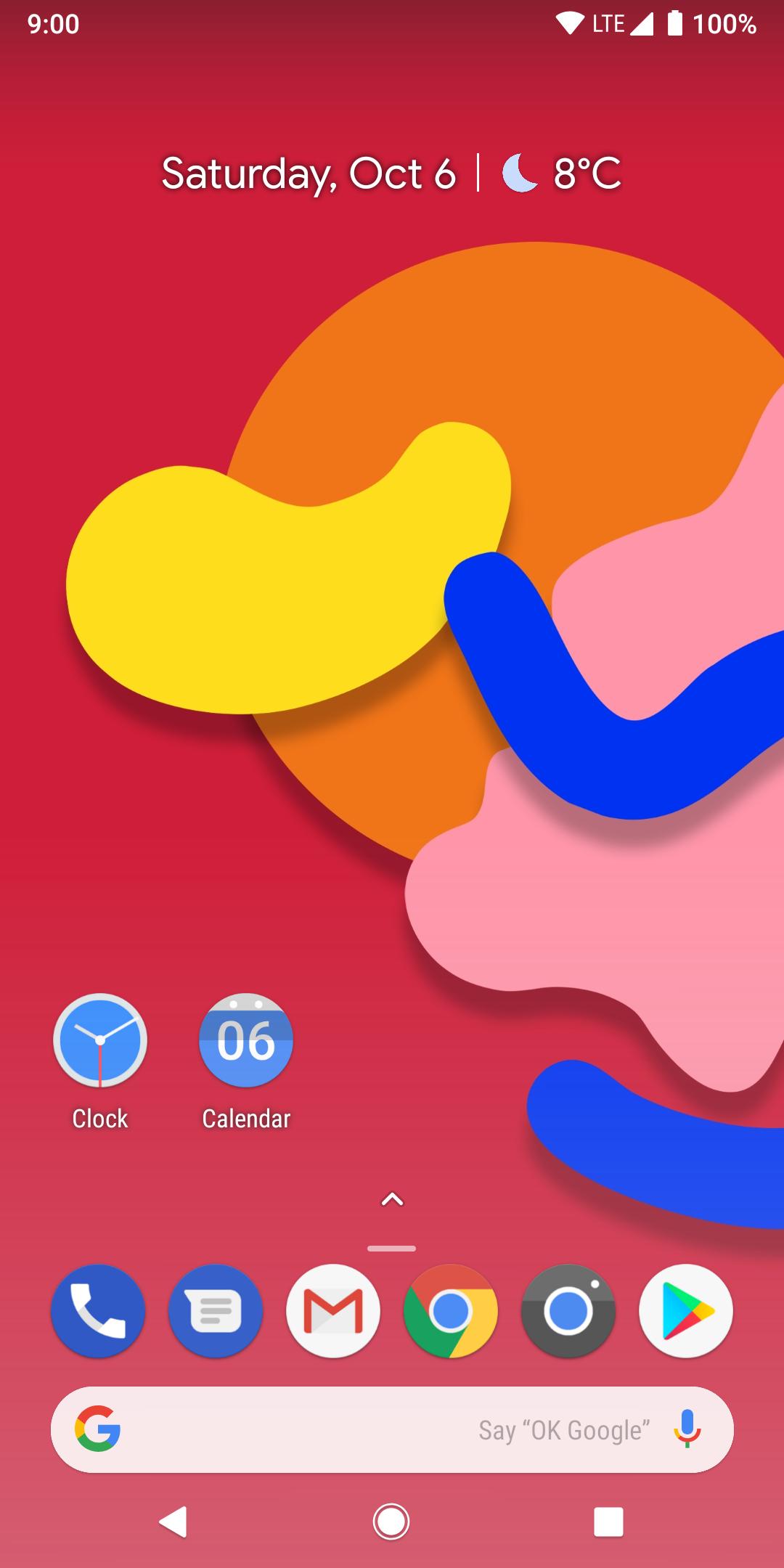The image showcases a cell phone screen with detailed status indicators and app icons. The top left corner displays the time as 9:00, while the battery icon shows a full charge at 100%. The connectivity indicators include a fully white Wi-Fi symbol and the LTE network label. The phone's home screen also displays the date as Saturday, October 6, and the current temperature as 8 degrees Celsius.

The wallpaper features a vibrant, abstract design with a dominant red background, complemented by an orange oval shape. Additionally, there are dynamic squiggly lines colored in yellow and blue.

Prominent app icons on the home screen include the Calendar app, the Clock app, and the Google Play Store app. The Google Chrome icon is also visible. A Google Search bar is present, featuring a recognizable microphone icon for voice searches. At the bottom of the screen, there is a circular home button.